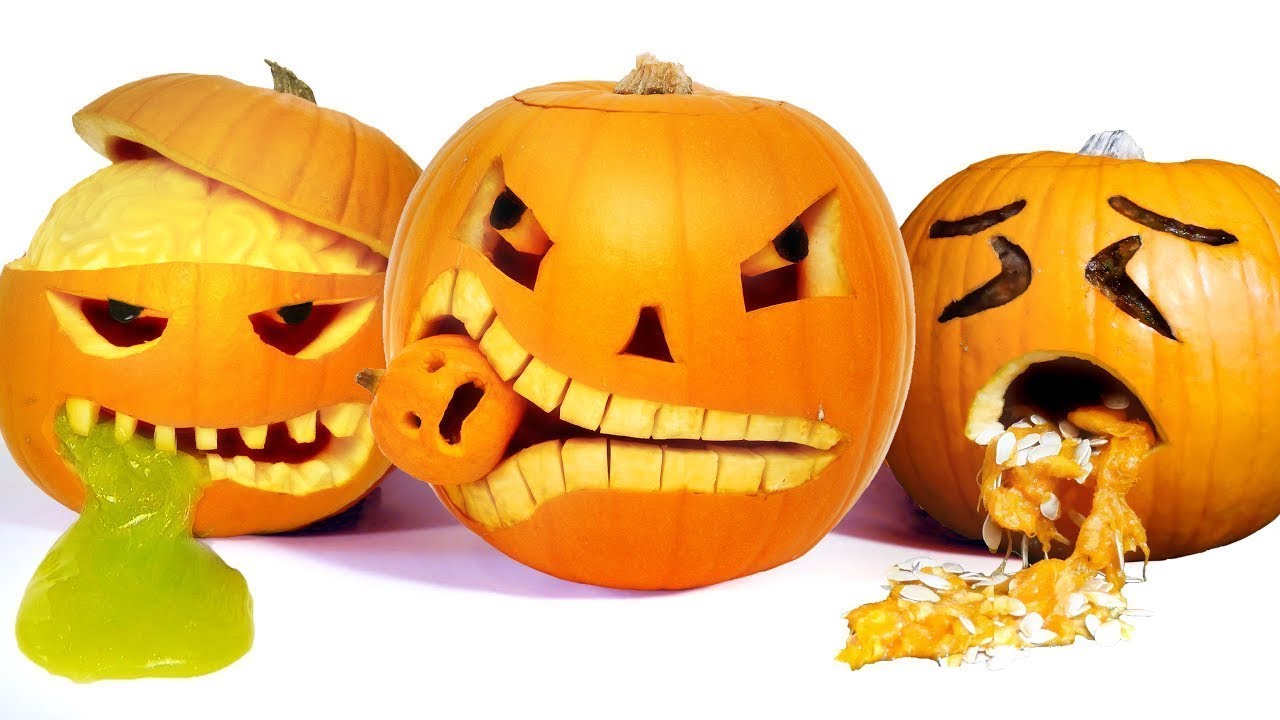The image depicts three meticulously carved jack-o'-lanterns, each showcasing a unique and imaginative design. Positioned in the center, the largest pumpkin features an ominous expression with jagged teeth and appears to be in the process of devouring a smaller jack-o'-lantern, which it holds between the exaggerated widening of its mouth. Its eyes are dark and malevolent, adding to its sinister demeanor. To the left, a slightly smaller pumpkin is presented with its top removed, exposing what looks like a carved brain inside. This pumpkin has cat-like eyes made from inserted materials resembling berries, teeth that resemble fangs, and green slime oozing from its mouth, enhancing its grotesque appearance. The smallest pumpkin on the right adds a touch of humor and horror, with its eyes closed in apparent distress as it vomits its insides, including seeds and orange pulp, in a dramatic display of pumpkin “guts” spilling out. The detailed carvings, from the green goo to the embedded eyes, showcase a high level of craftsmanship and creativity.